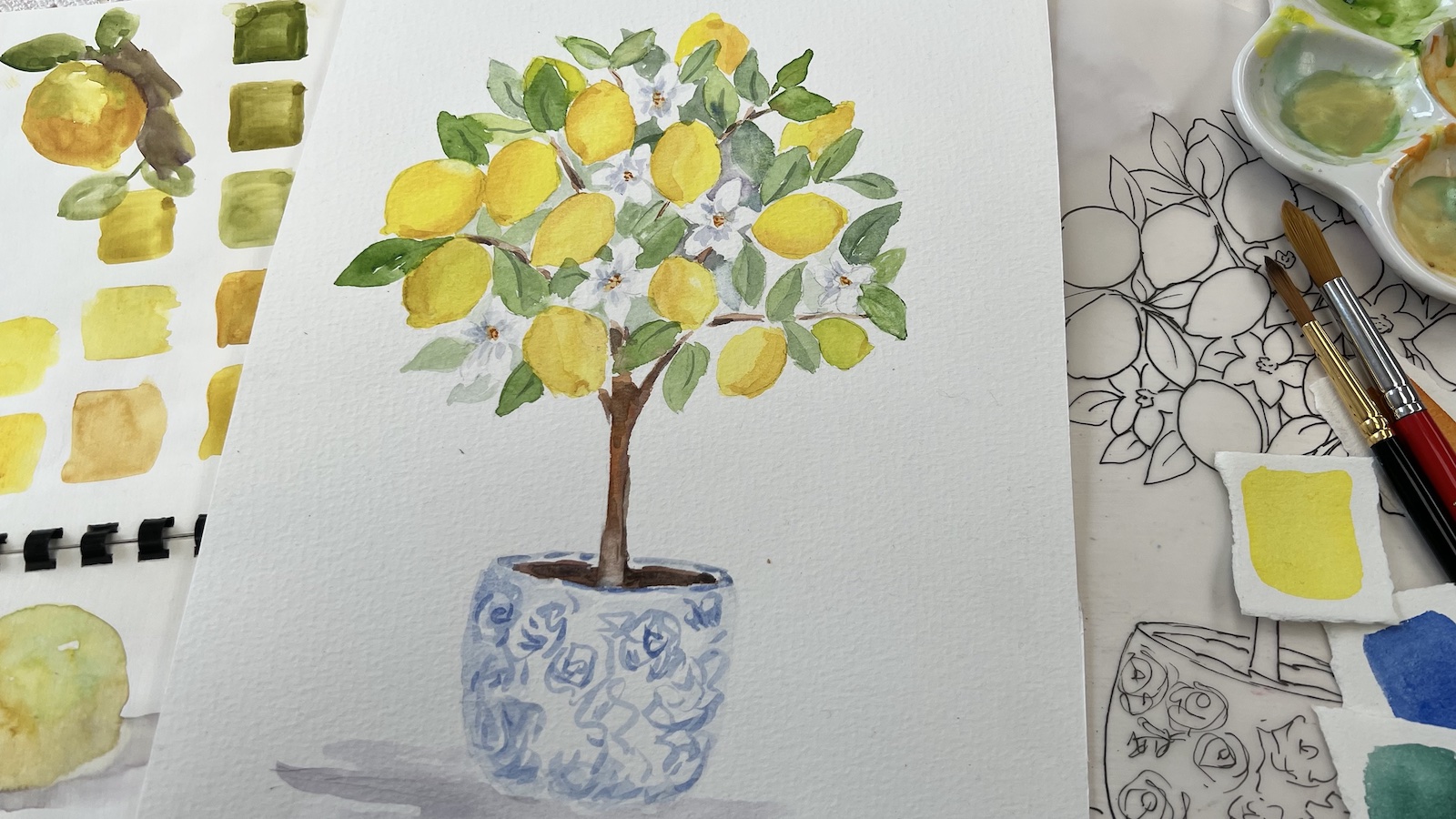In this photograph, a white canvas fills the center, dominated by a detailed watercolor painting of a lemon tree. The tree sprouts from a blue and white pot with intricate designs, its brown stem supporting an array of vibrant green leaves, numerous yellow lemons, and a scattering of delicate white flowers. The painting occupies the majority of the canvas, which extends slightly rightward and upward, and also off the bottom of the image. Surrounding the main artwork are various artistic tools and other drawings. To the right, two paintbrushes extend outward, paired with a pencil sketch of the same lemon tree and pot. Further to the right, small squares of painted color patches—yellow, blue, and green—can be seen. The upper right corner also features a paint-mixing tray that partially exits the frame. On the left side of the canvas, there is a black-bound notebook displaying swatches of paint colors and a painted fruit. Nearby, some additional swatches and round shapes are visible, suggesting ongoing experimentation and practice. The scene captures a rich, detailed snapshot of an artist's workspace, brimming with tools, sketches, and the vibrant central watercolor painting.